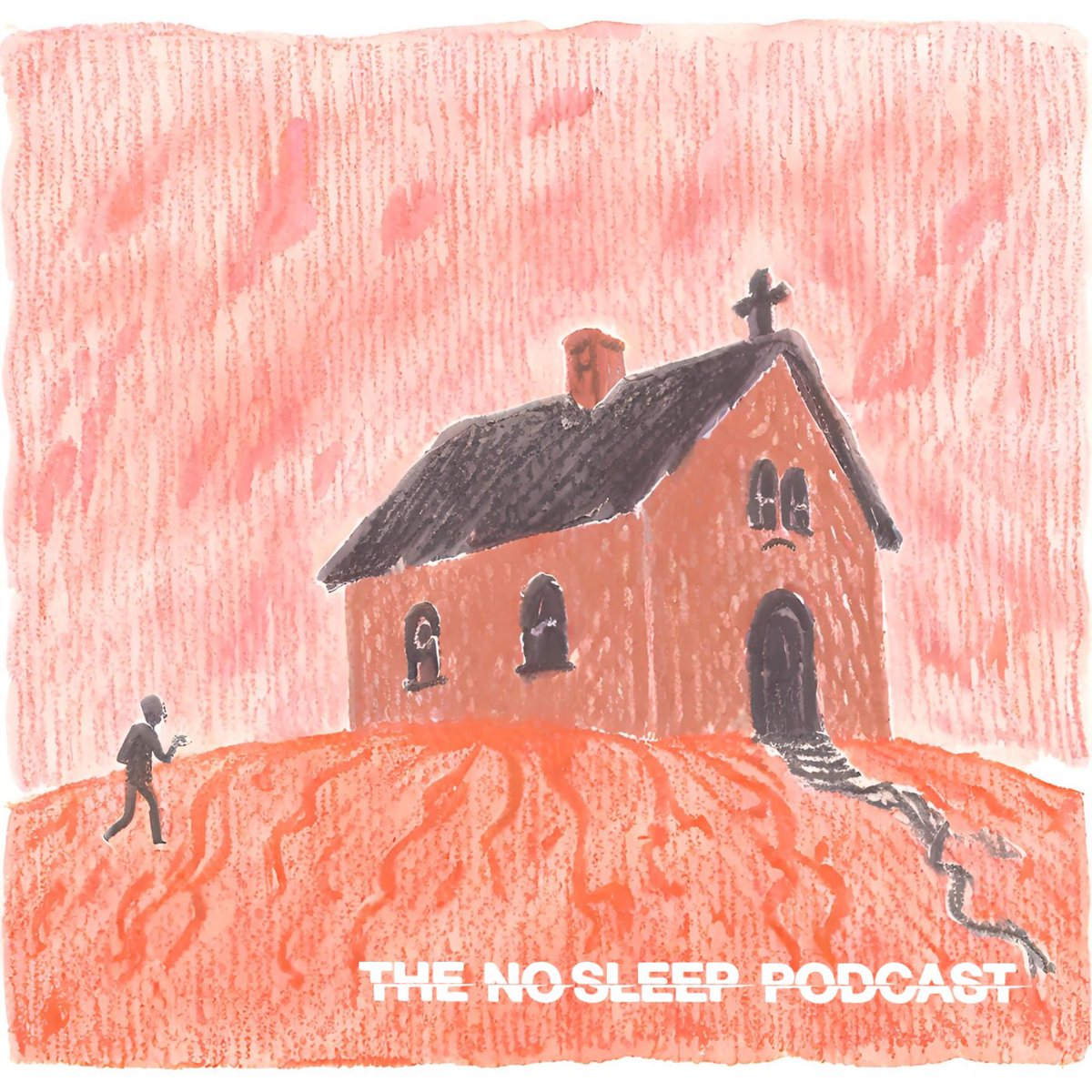The image is reminiscent of an album cover, designed with a colored pencil style. Dominated by shades of red and black, the painting features a small church building set on a red hill. The church, identifiable by the black cross on its roof and a single chimney, has an open door with steps leading up to it and black windows. The sky and background are composed of reddish and pinkish-orange hues, creating a stark, eerie atmosphere. A black figure is depicted walking up a winding, squiggly path towards the church, enhancing the sense of an isolated journey. The overall composition includes various red vertical lines suggesting a turbulent environment. At the bottom of the painting, in white capital letters, the title "The No Sleep Podcast" is prominently displayed, using a distinctive font that adds to the intriguing and haunting feel of the artwork.